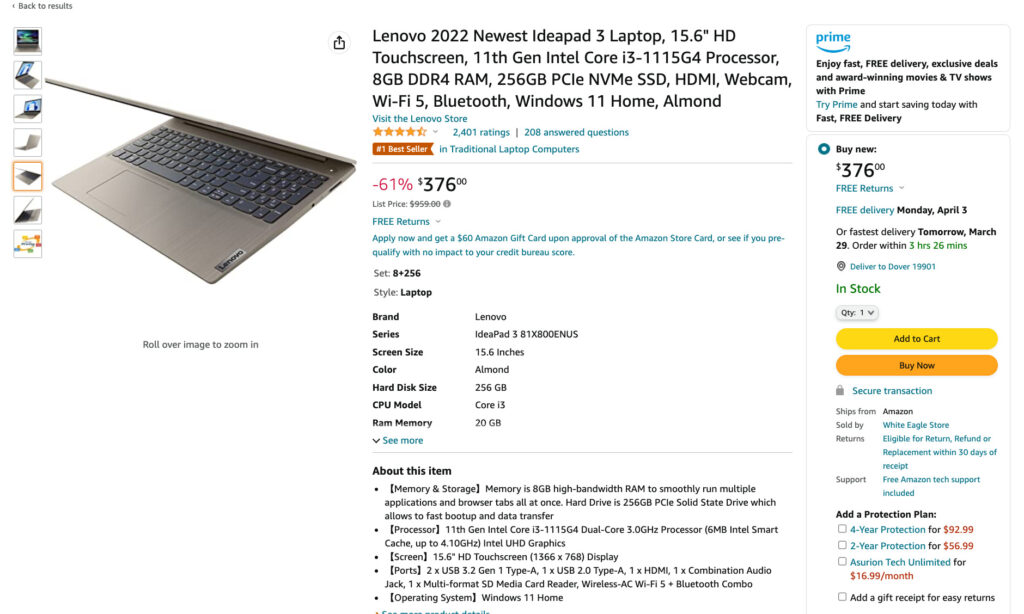This detailed caption describes a screenshot of an Amazon shopping page for the Lenovo 2022 Ideapad 3 laptop. The laptop features a 15.6-inch HD touchscreen and is powered by an 11th generation Intel Core i3-1115G4 processor. It includes 8GB of DDR4 RAM and a 256GB NVMe SSD, making it an efficient device for multitasking and fast data transfers. The device has an Almond color finish and offers connectivity options like HDMI, Wi-Fi 5, Bluetooth, and several ports, including two USB Type-A ports, a combination audio jack, and a multi-format SD card reader.

The Lenovo Ideapad 3 operates on Windows 11 Home and has received high customer acclaim, boasting a 4.5-star rating from 2,401 reviews and 208 answered questions. It is ranked as the number one bestseller in the traditional laptop computer category and is currently offered at a 61% discount, priced at $376, down from its original list price of $959. The item is eligible for free returns and offers a promotional $50 Amazon gift card upon approval of an Amazon Store Card. Additionally, the laptop comes with a promo application that does not impact the user's credit bureau score.